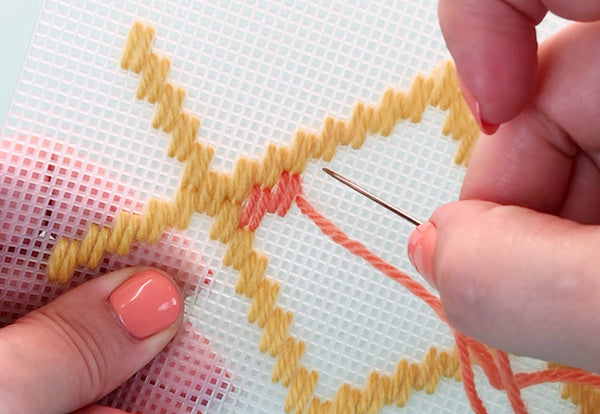In this close-up image, a lady is engaged in needlework, holding a piece of plastic cross-stitch mesh with intricate details. Her hands dominate the frame, showing only the fingers and the thumb, each fingernail painted in a peachy-orange hue. The right hand grasps a needle threading orange-colored floss, while the left hand stabilizes the mesh, characterized by its tiny, diamond-shaped holes. Already visible are golden yellow threads forming small diamond patterns. The lady appears to be in the process of filling in one of the squares with the orange thread, against a plain white backdrop, likely a desk or tabletop, devoid of any other distinguishing features.